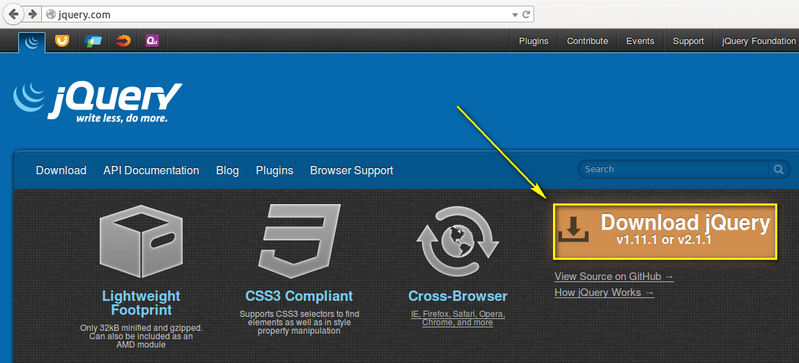The image showcases a web page themed primarily in blue and gray, featuring the jQuery logo prominently, with "jQuery" rendered in white. The 'Q' in 'jQuery' is capitalized, accompanied by the slogan "Write Less, Do More," also in white. Below the logo, navigation options include "Download," "API Documentation" (with "API" capitalized), "Blog," "Plugins," and "Browser Support." There's a search bar with a magnifying glass icon at the top.

The URL bar displays "jQuery.com" alongside a globe icon and a left-pointing white arrow. The main content of the page has a gray background and features text highlighting jQuery's "lightweight footprint," its compliance with "CSS3," and its "cross-browser" capabilities.

An orange rectangle in the center includes a black download icon—a half square with an arrow—and text in white stating "Download jQuery v1.11.1 or v2.1.1." This orange rectangle is bordered by a yellow rectangle, from which a yellow arrow points at the orange rectangle. Additionally, there are two labels with arrows pointing to the right: one reads "View Source on GitHub," and the other says "How jQuery Works."